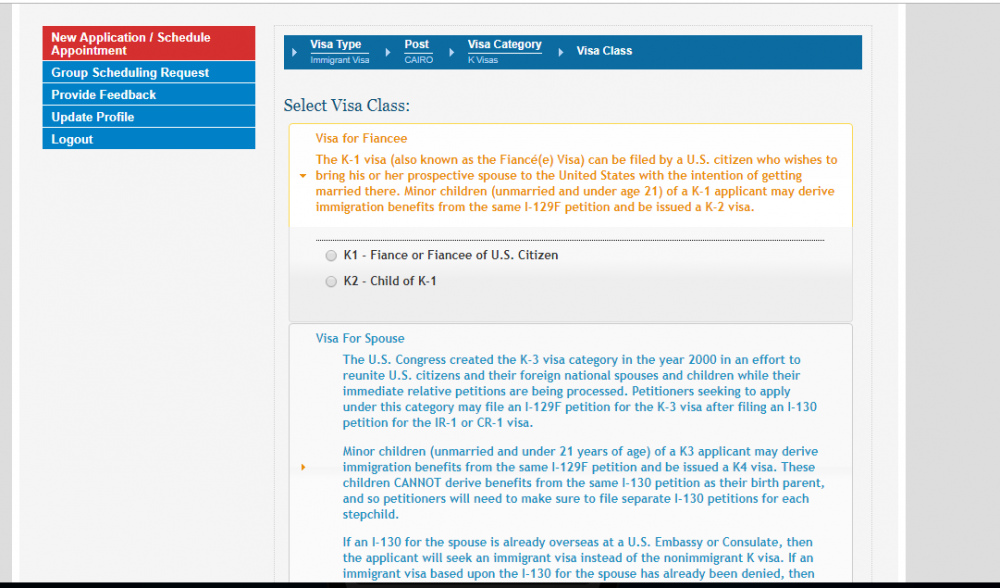Sure, here is a cleaned-up and detailed caption for the image described:

---

The image captures a section of a website with a predominantly gray background and an assortment of font colors. 

On one side of the image, there is a multi-colored box divided into a red section and a blue section. The red section, with white font, reads "New Application / Schedule Appointment". The blue section contains various instructions also in white font which include "Group Scheduling Request," "Provide Feedback," "Update Profile," and "Log Out".

On the other side of the image, a thin navy bar displays in white text detailing visa information: "Visa Type: Immigrant Visa," "Post: Cairo," "Visa Category," "Visa Class". Below this, a navy section prompts the user to "Select Visa Class," and in an orange highlight, it mentions "Visa for Fiancé." This section explains that the K-1 Visa, commonly referred to as the fiancé visa, allows a U.S. citizen to bring their prospective spouse to the United States with marriage intentions. It also highlights that minor children (unmarried and under 21) of a K-1 applicant can derive immigration benefits from the same I-129F petition and qualify for a K-2 Visa.

Further down, black text outlines two radio buttons: one for the K-1 Fiancé(e) of U.S. Citizen and another for the K-2 Child of K-1. Below, in blue text, it elaborates on the K-3 Visa for Spouses. This visa category was created by the U.S. Congress in 2000 to help reunite U.S. citizens with their foreign national spouses and children while their immediate relative petitions are processed. It specifies the filing requirements for petitioners seeking this category, stating that they can file an I-129F petition for the K-3 Visa after filing an I-130 petition for the IR-1 or CR-1 Visa. Minor children (unmarried and under 21) of a K-3 applicant may derive immigration benefits from the same petition and qualify for a K-4 Visa. It also notes the need to file separate I-130 petitions for each stepchild, as benefits cannot be derived from a single I-130 petition.

The description of the process for applicants whose I-130 for the spouse is already at a U.S. embassy or consulate ends abruptly: "If an immigrant visa based on the I-130 for the spouse has already been denied then…"

---

This detailed caption provides a clear, organized, and comprehensive overview of the website captured in the image.